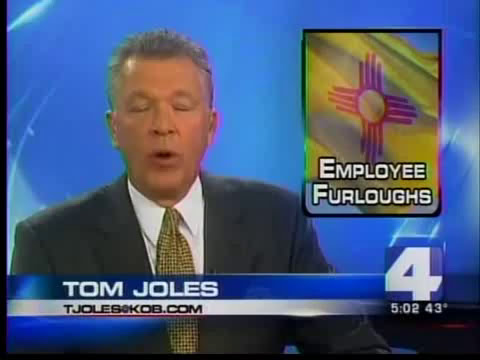This screenshot captures a TV news segment featuring a male news anchor with short gray hair, seated against a blue patterned background. The anchor, appearing to speak mid-sentence, has his eyes closed and mouth slightly open. He is dressed formally in a dark gray suit paired with a white dress shirt and a distinctive yellow tie adorned with black dots. To the right of the anchor, a rectangular graphic has been superimposed, displaying the New Mexico flag—a yellow backdrop with a red circle and four red lines extending outward—accompanied by the text "employee furloughs." Below the anchor, a horizontal banner presents his name, "Tom Joles," in white letters on a blue strip, followed by his email "TJOLES at KOB.com" in black text on a white strip. In the bottom right corner, the channel logo, featuring the number 4, is displayed above a numeric figure reading "502.43 degrees."